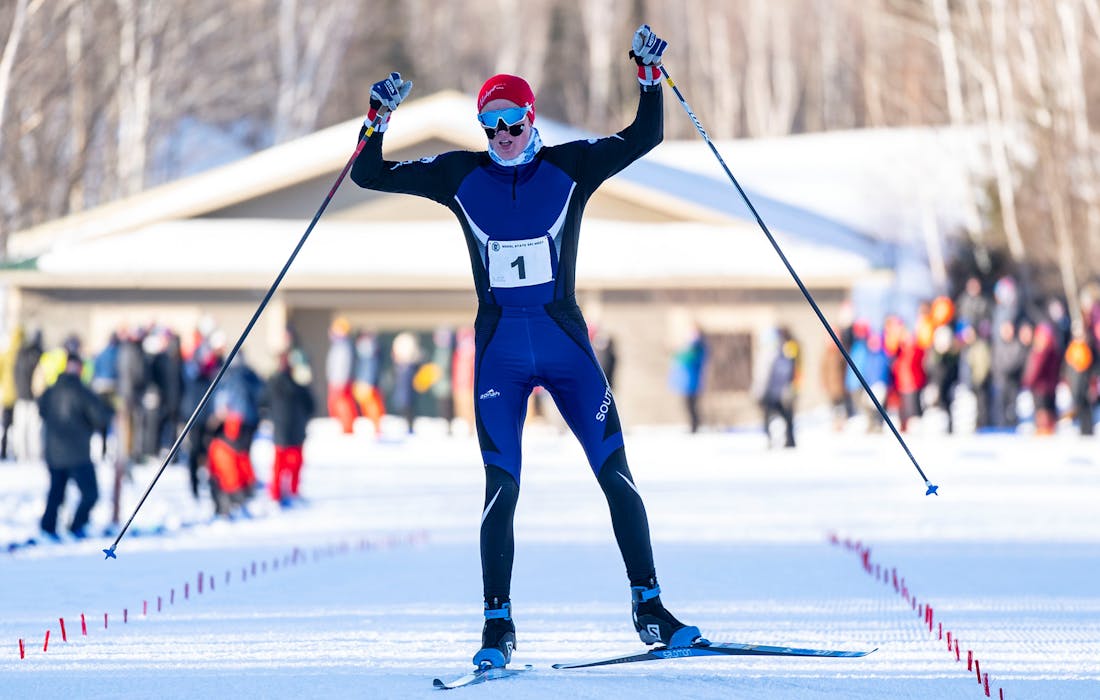A high-quality image captures a cross-country skier crossing the finish line with his arms outstretched in triumph, ski poles extended in each hand. He wears a red hat, iridescent blue-tinged sunglasses, and a dark blue and black ski suit that covers him from neck to feet. A white plaque on his chest prominently displays the number one. The skier stands on an icy, snowy surface marked by small orange tags on both sides. In the background, a cheering crowd adds to the celebratory atmosphere.